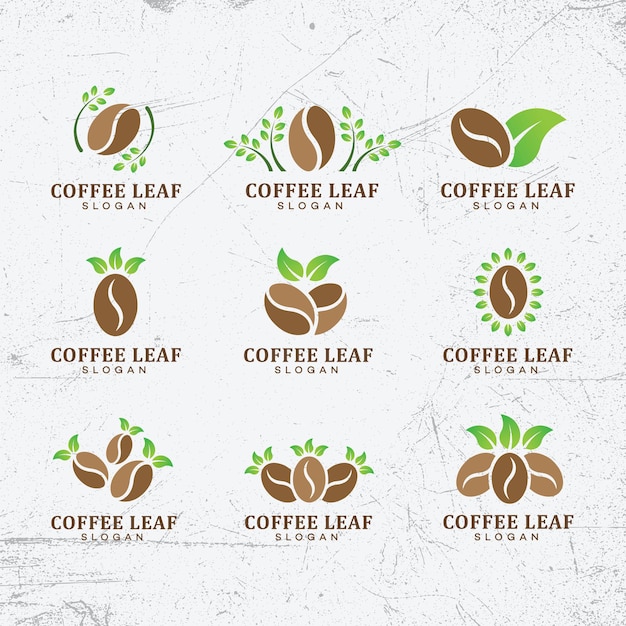This photo showcases a sheet of design samples for a coffee company, prominently featuring nine distinct logo variations arranged in a 3x3 grid. Each logo consistently displays the "Coffee Leaf" title in uppercase brown letters with a matching slogan beneath it. The primary element in each design is a brown coffee bean, varying in shades from light to dark brown, accentuated with green leaves. The top row's first logo depicts a single coffee bean encircled by curling leaves, while subsequent designs alter the arrangement of the beans and the positioning of the leaves—some leaves stretch outward, some are solid, and others form miniature clusters. The background of the sheet is light gray, marred by dark gray and black smudges and lines, adding a textured appearance. This gives the backdrop a slightly worn look, with identifiable smudging concentrated in the corners and fine lines traversing its surface.